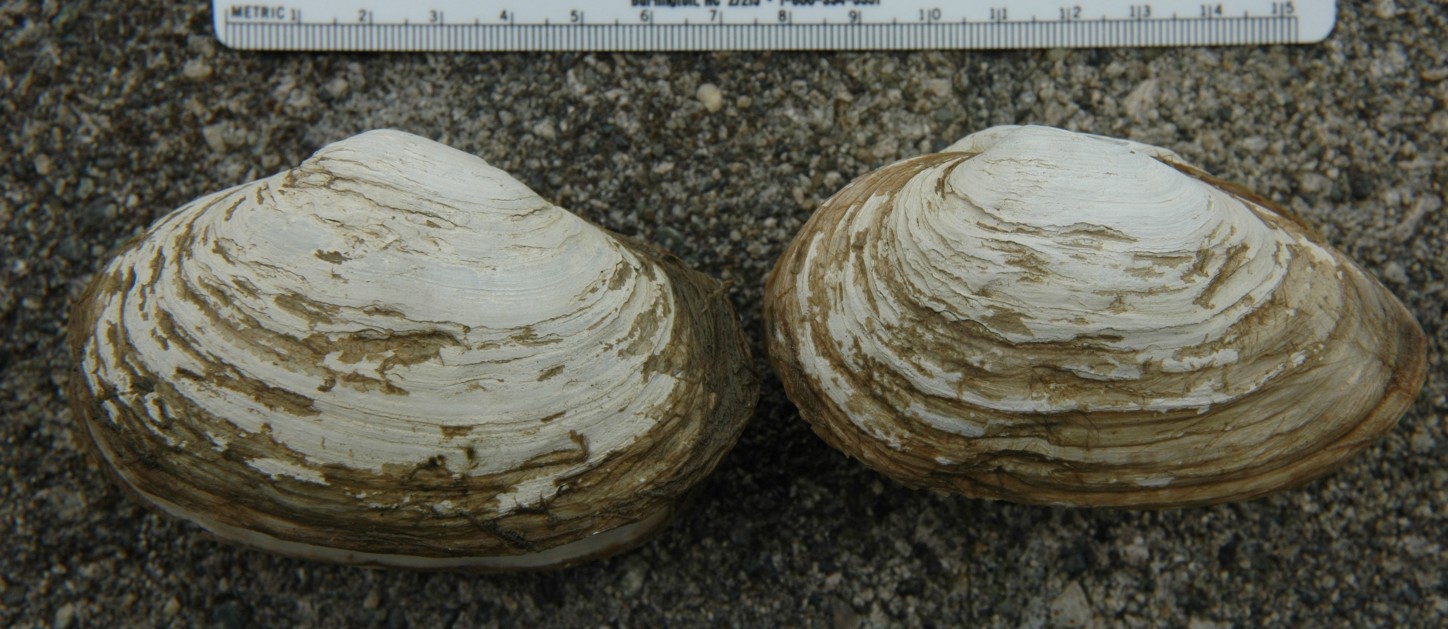The photograph captures two closed clamshells or oysters, side by side, on a ground that appears to be either a concrete surface or compacted sand interspersed with black and gray pebbles. The white and brown shells, adorned with several ridges and lighter colored striations, are centered in the image. Above the shells, a white plastic metric ruler stretches horizontally, measuring from 0 to 15 centimeters. The shells vary slightly in hue, with the left being a darker brown and the right a lighter tan. The lighting is neutral, casting slight shadows beneath the shells, and the overall scene has a natural, earthy tone with shades of white, tan, brown, and touches of black.